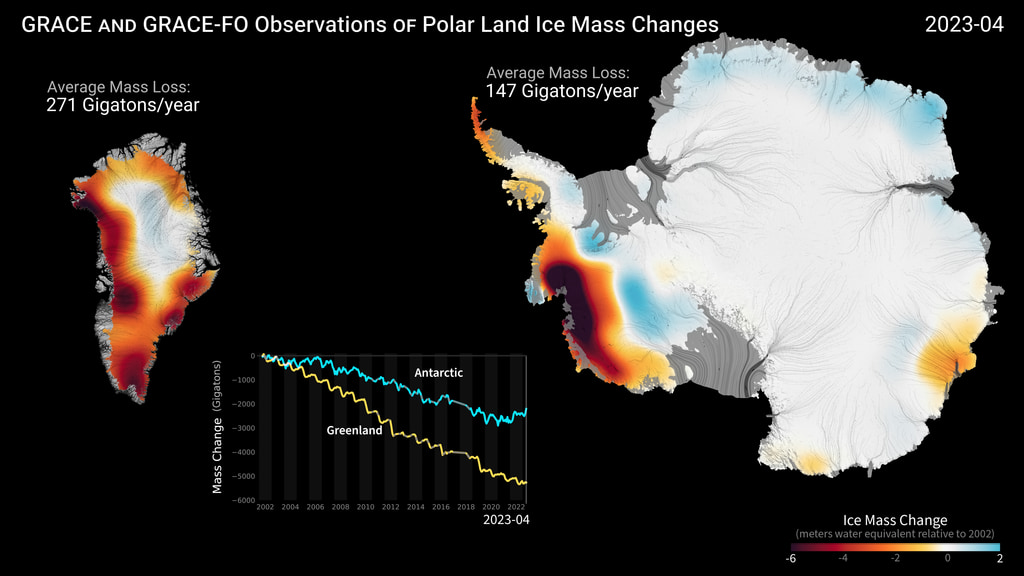The rectangular image features a black background and lacks a border. In white text in the upper left corner, it reads "GRACE and GRACE-FO Observations of Polar Land Ice Mass Changes," with "2023-04" marked in the upper right. On the left side, the caption "Average mass loss" is printed in gray, followed by "271 gigatons per year" in white. Below this is a topographic map depicting Greenland, showing a white center with orange and brown edges indicating mass loss.

Adjacent to this, a graph is present with an x-axis spanning from 2002 to 2022 and a y-axis indicating mass change in gigatons. Two descending lines are depicted: a yellow one for Greenland, showing a steeper decline, and a blue one for Antarctica. The graph highlights the differing rates of ice mass loss in these regions.

To the right of the graph is a larger topographic map, identified as Antarctica, labeled "Average mass loss: 147 gigatons per year." This map also shows a predominantly white center with peripheral coloration indicating various degrees of ice mass change, transitioning from blue to orange and brown tones. In the lower right corner, a color bar key explains the correlation between the colors and the degree of ice mass change, with darker orange and brown representing higher loss and white and blue representing lower loss.